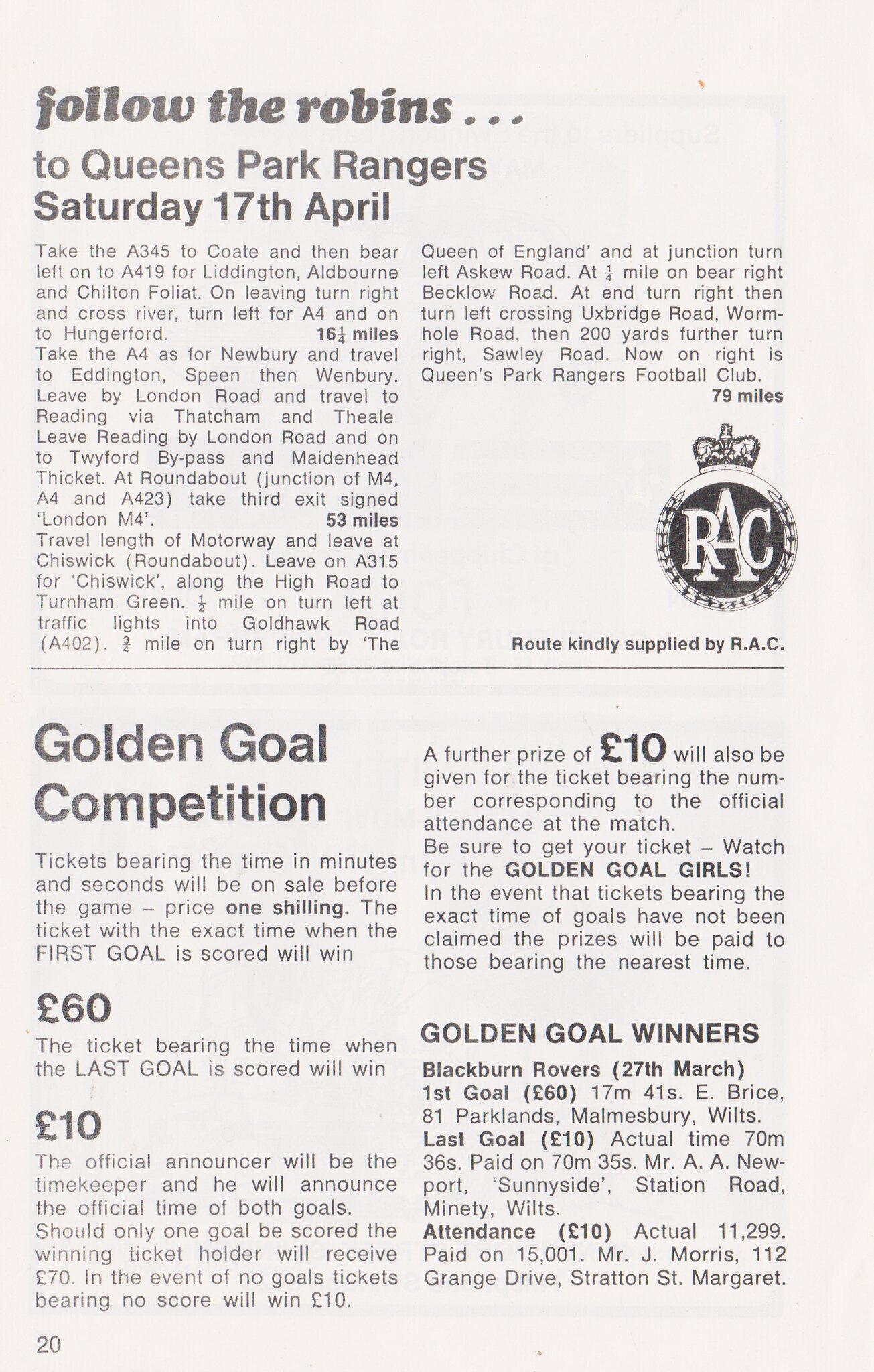This is a black-and-white newspaper or newsletter clipping, likely from the sports section, exhibiting two distinct articles stamped as page 20. The upper half features the article titled "Follow the Robins to Queens Park Rangers, Saturday, 17th April." Set in bold, lowercase letters, this section provides detailed route instructions for traveling to Queens Park Rangers, entailing a 16.25-mile journey starting from A345 to Colton, then left onto A400 towards Littleton, Epburn, and Chitton Foliage, before finally turning right at Close River and left onto A4 towards Hungerford. This section also sports a circular logo in the lower right corner featuring the letters "RAC" encasing a large 'A' flanked by an 'R' and 'C,' topped with a crown, attributed to the Royal Automobile Club.

The bottom half highlights the "Golden Goal Competition," describing a contest where tickets bearing the time in minutes and seconds are sold for one shilling. The competition awards £60 for the first goal, £10 for the last goal, and an attendance prize of £10. Detailed instructions on prize distribution are included, such as provisions for ties and unclaimed prizes. Additionally, past winners are listed, including Golden Goal winners from Blackburn Rovers on March 27th, with specific goal times and winners' names and locations provided. The page's print bleeds through slightly from the other side, hinting at its vintage magazine origin, though the exact publication remains unidentified.